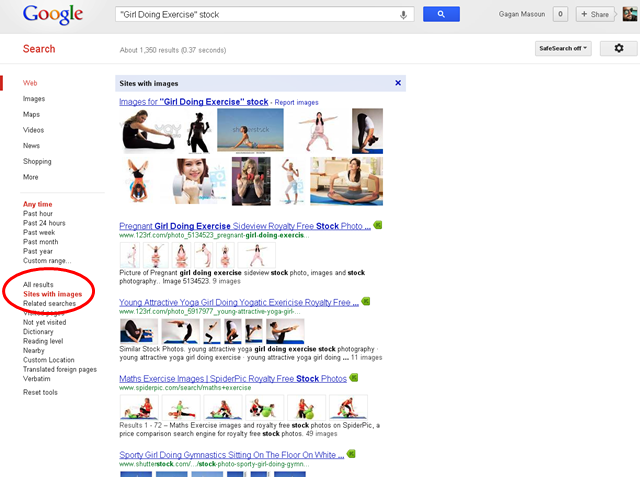The image shows a Google search page. In the upper left corner, the familiar Google logo appears in its traditional colored letters—blue, red, yellow, and green. Centered on the screen is the search bar, which contains the phrase "girl doing exercise stock" with the exact phrase "girl doing exercises" in quotation marks. To the right of the search bar, there is a blue search button.

Directly below the logo, the word "Search" appears in red, followed by several filter options: "Web" (highlighted in red, indicating the current selection), "Images," "Maps," "Videos," "News," "Shopping," and "More." Underneath these options, another filter presents a dropdown menu titled "Any time," offering further refinements such as "Past hour," "Past 24 hours," "Past week," "Past month," "Past year," and "Custom range." An additional filter labeled "All results" offers choices like "Sites with images" and "Related searches."

A red circle, added using a photo editor, highlights the options under "All results" and "Sites with images." Below these filters, a series of image search results titled "Images for girl doing exercise stock" is displayed. There are two rows, each containing five images.

The first search result caption reads "Pregnant girl doing exercise, side view, royalty free, stock photo." The following captioned image is titled "Young attractive girl doing exercise, yoga, yogaistic exercise, royalty free."